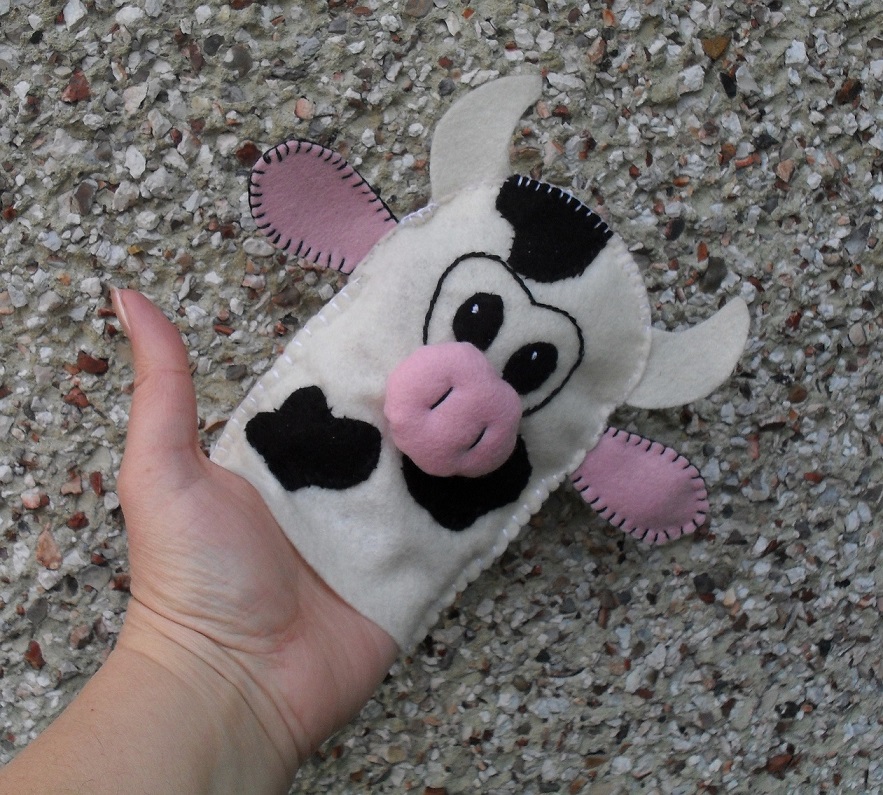The image features a handmade, stitched hand puppet designed to resemble a cow’s head. The puppet, which appears to be DIY, fits over the four fingers of a human hand, leaving the thumb exposed. The cow head puppet, predominantly white with black spots, showcases a large pink nose, pink ears with black stitching, and two white horns protruding from the top. Its cartoonish eyes, outlined with black stitching, add to its whimsical appearance. The puppet is set against a neutral-colored stone or marble countertop, featuring shades of white, gray, and brown. The visible details and careful stitching suggest a crafted, playful depiction of a cow.